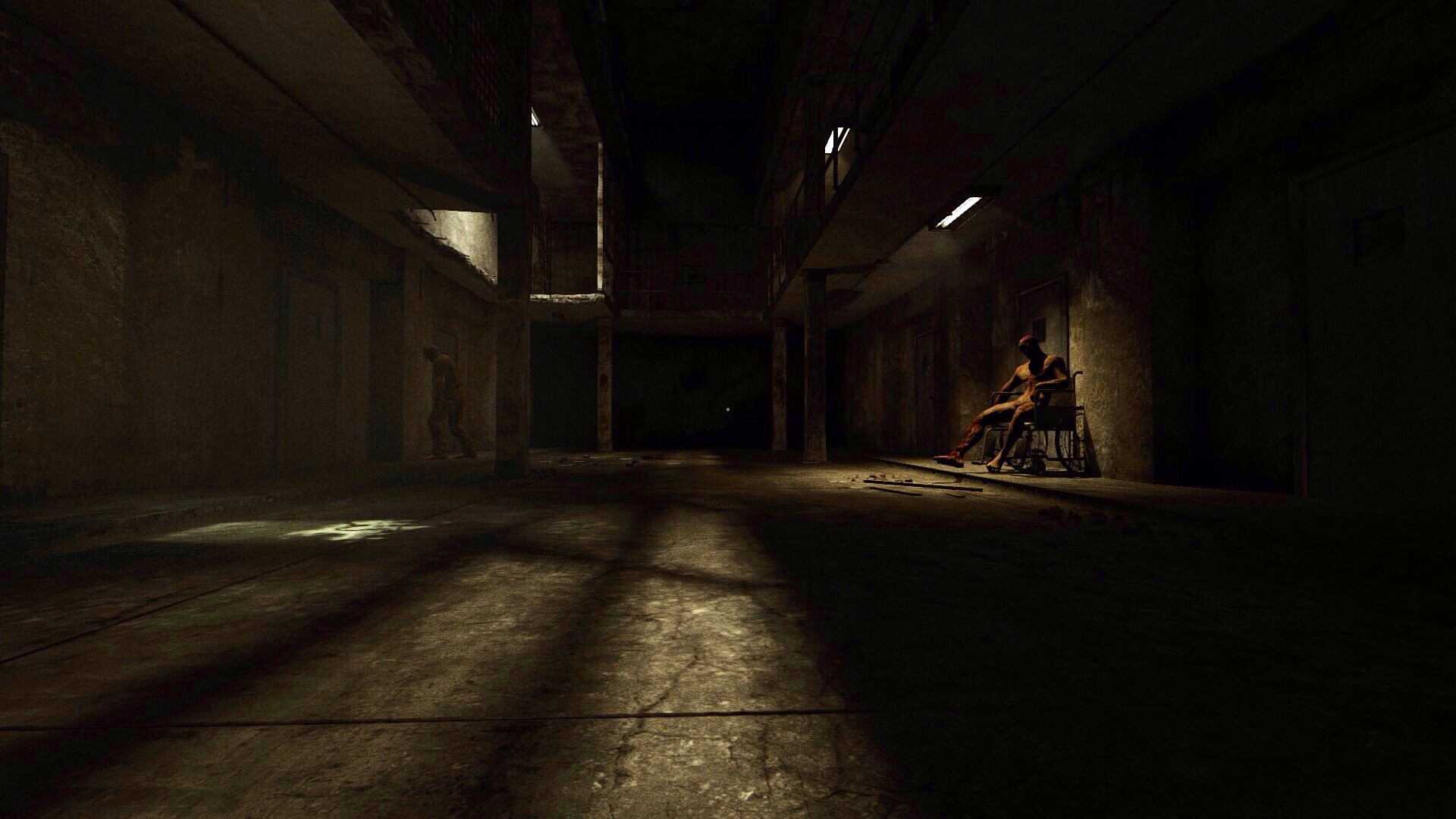The image appears to be a dark industrial or prison-like facility, possibly from a video game, depicting a dilapidated concrete hallway. The scene is minimally illuminated by a few flickering fluorescent tube lights, casting weak shadows on cracked concrete floors and columns. In this multi-level enclosure, the decrepit environment is accentuated by the presence of two eerie characters: one zombie-like figure is shuffling forward in a state of distress, while another character, seemingly only dressed in shorts and sandals, is seated in a wheelchair with a despondent posture against a building's wall. Shadows loom heavily across the scene, amplifying the sense of abandonment and decay.